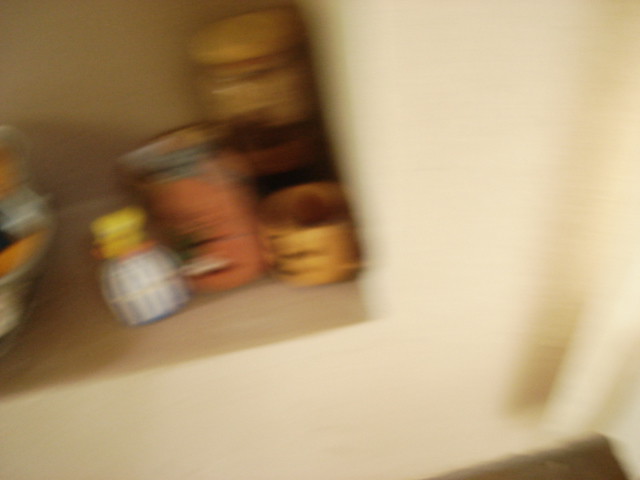This image is a very blurry photo of a small shelf built into a white drywall. The shelf, which seems to be part of a cabinet or cupboard setup, holds various items that are difficult to clearly identify due to the motion blur. There are several containers: a salt shaker, a small yellow canister, a can resembling a short 4-ounce tomato sauce can with a gold lid, a can with an orange label potentially depicting a coconut, a bottle of lemon juice, and another jar with a yellow lid in the back. The shelves are filled, but the blurred nature of the photo makes it hard to discern all the details clearly.